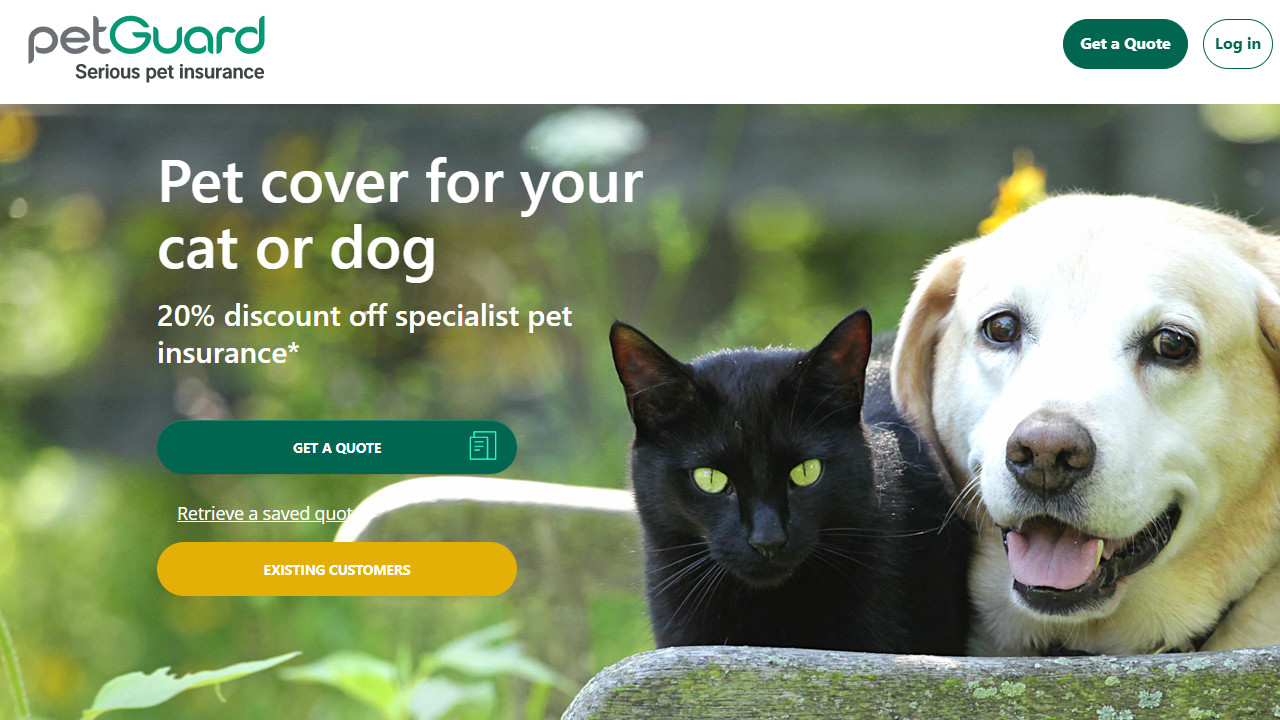On this website for Pet Guard Serious Pet Insurance, the layout is designed with user convenience in mind. Along the left side of the screen, there is a green button labeled "Get a Quote" in white lettering, followed by a white button labeled "Log In."

At the top of the page, the Pet Guard logo is prominently displayed, with the tagline "Serious Pet Insurance" situated just below it. Directly beneath this tagline is a box featuring a striking image of a pair of pets: a white Labrador Retriever with a black nose and a hint of a pink tongue, and a completely black cat with vividly bright yellow eyes. Both animals are attentively staring at the photographer.

Within this box, white text reads, "Pet Cover for Your Cat or Dog," immediately followed by an enticing offer: "20% Discount off Specialized Pet Insurance." Right below this, another green button invites visitors to "Get a Quote." Further down, additional service options are listed: a link to "Retrieve a Saved Quote" and a section specifically for "Existing Customers," which includes a prominent yellow button for easy access.